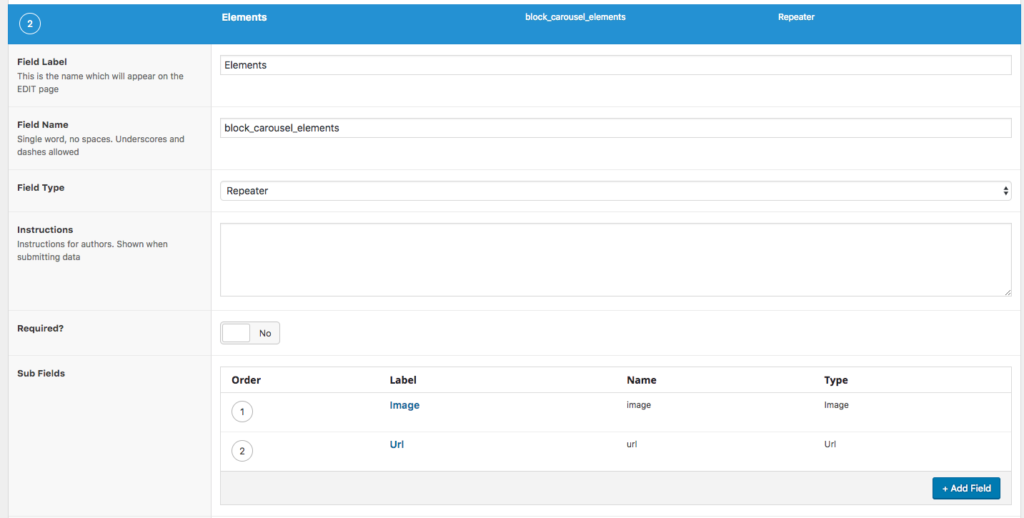This is a detailed description of an image captured from a computer or smart device screen. The image is displayed horizontally from left to right. At the very top, there is a long, blue rectangular strip. On the upper left-hand side of this strip, a white circle contains the number "2". Moving towards the right along the strip, the words "elements," "black carousel elements," and "repeater" are visible.

On the left side of the screen below the strip, there is a gray box arranged vertically. This box has several headings in bold – "Field Label," beneath which the text "This is the name which will appear on the edit page" is displayed. Another bold heading reads "Field Name,” instructing that this should be a single word with no spaces, though underscores and dashes are allowed. Additional bold headings include "Field Type," "Instructions," with a note below it stating "Instructions for authors is shown when submitting data," and "Required?" with subfields in bold.

To the right of this gray box, the background appears white. There’s a sequence of boxes interspersed with white spaces. The first box contains the word "elements." After a white space, the next box reads "black_carousel_elements." Another white space follows before a box that says "repeater." Following more white space is an empty box, and then a box with an unchecked option labeled "no.”

At the very bottom of the screen, there is an organized area where the headings "Order," "Label," "Name," and "Type" are displayed in bold. Under the "Order" heading, the numbers "1" and "2" are listed. Under the "Label" in blue are the words "image" and "URL." Correspondingly, "image" and "URL" are listed in black under both the "Name" and "Type" headings.